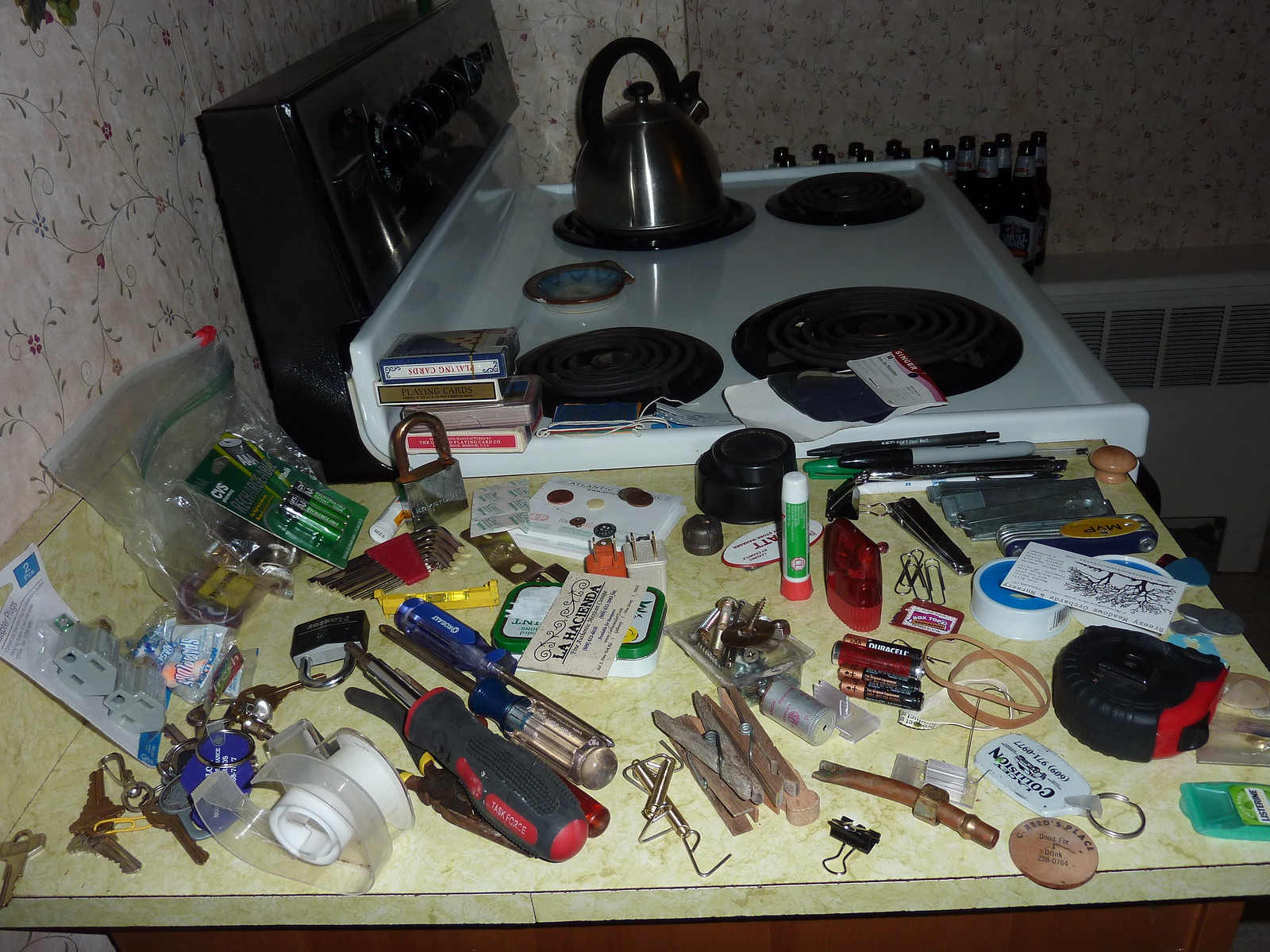The image captures a cluttered kitchen scene. At the top of the photograph, a stove with four burners is prominently featured, with a stainless steel teapot resting on the top left burner. Below the stove, the countertop is in complete disarray, as if an entire junk drawer has been emptied onto it. The yellow countertop is covered with a jumble of items, including wooden clothespins, screwdrivers, various kinds of tape, a tape measure, Duracell batteries, Krazy Glue, and an assortment of small tools. There are also binder clips, pocket knives, nail clippers, markers, pencils, additional batteries, multiple keys, and master locks scattered across the surface. The chaotic spread provides a snapshot of an everyday kitchen cluttered with miscellaneous household items.